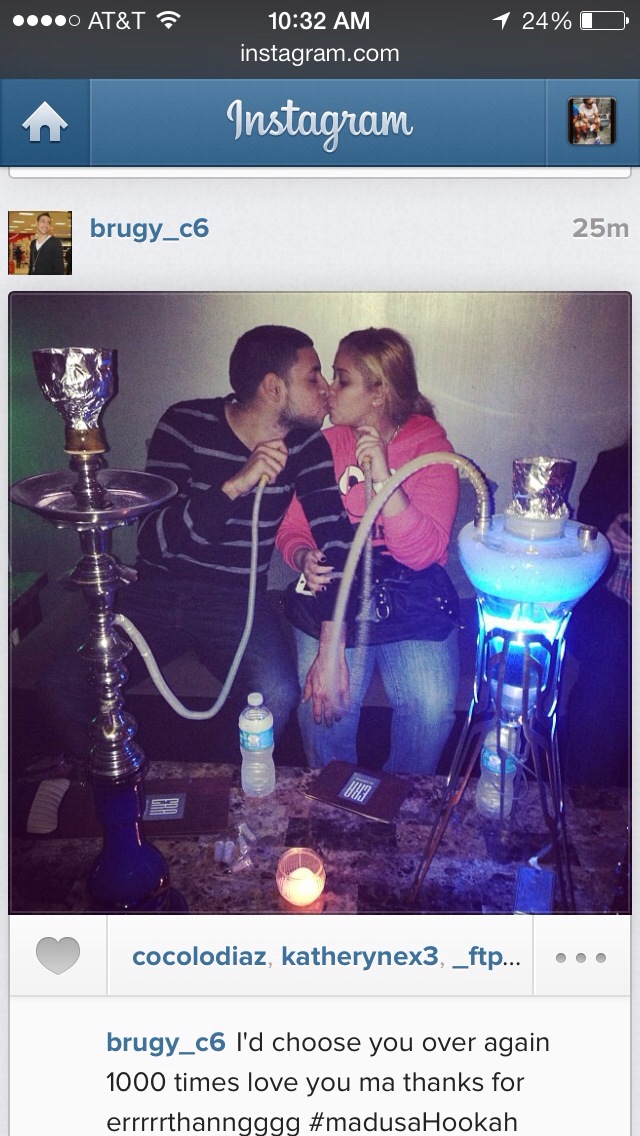The image is a detailed screenshot from a cell phone displaying an Instagram post. At the top of the screen, there is a dark gray header bar. On the left side of this bar, five circles indicate the signal strength with four of them filled. Next to it, in white text, it says AT&T, and in the center, it displays the time 10:32 AM with "Instagram.com" written in smaller white text below. To the right, the battery icon shows 24% remaining. Directly beneath this header, a blue banner stretches across the width of the screen with the word "Instagram" written in cursive font in the center.

Below the banner, the post begins with a small circular profile picture to the left labeled as "broogie_C6" in blue text. To the right of the username, it indicates "25 minutes" in gray text. The main image below the username is a vibrant color photograph of a couple seated and kissing, each holding a hookah pipe, with large hookah vases visible in front of them. The background behind the couple features a whitish wall.

Following the photograph, the username "broogie_C6" appears again in blue text, followed by the caption in black: "I'd choose you over again a thousand times. Love you Ma. Thanks for everything. #MedusaHookah."